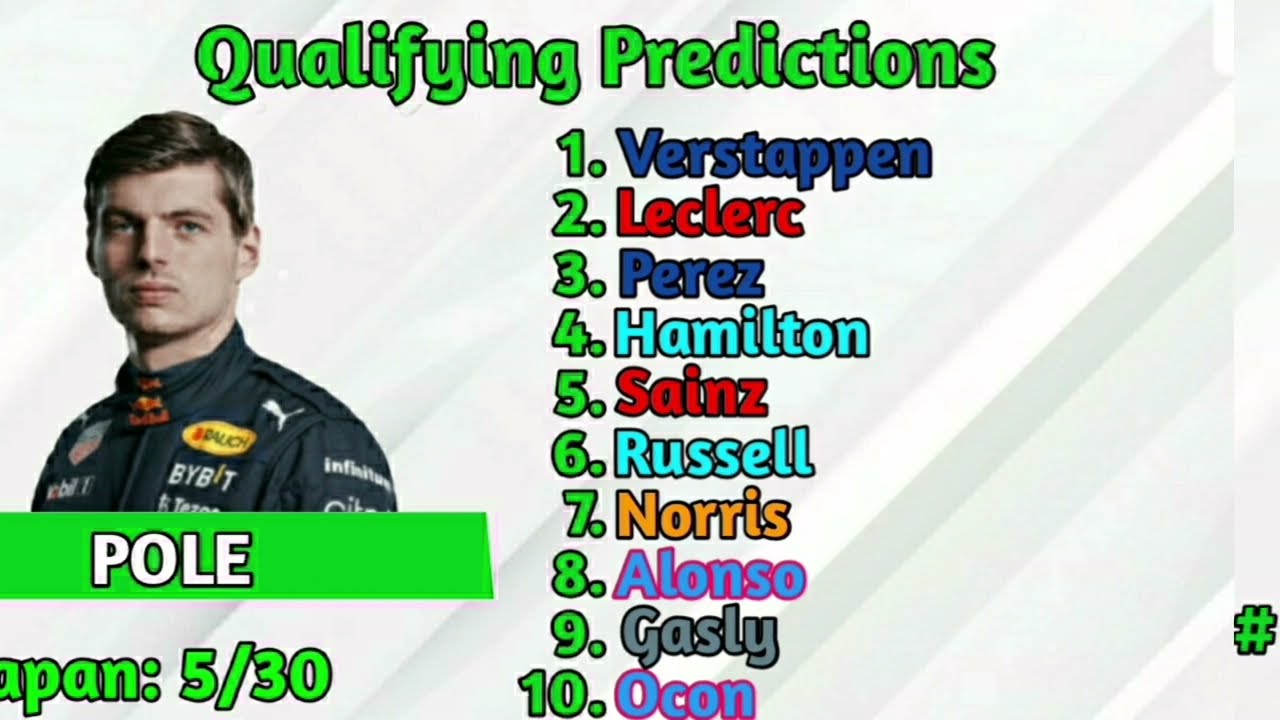The image features a detailed graphic of sports statistics prominently displayed on the right side. On the left, there is a head-and-shoulders photograph of a white man with short, blondish-brown hair and a serious expression, dressed in a racing suit adorned with various corporate logos including a prominent Puma logo. Below his image, a narrow green rectangle features the word "POLE" in bold, white uppercase letters, with the text "Japan 5/30" in green below it.

At the top of the graphic, "Qualifying Predictions" is written in a bright, neon green, bubbled font. Below this heading is a numbered list ranking ten names:
1. Verstappen (in navy blue)
2. Leclerc (in red)
3. Perez (in navy blue)
4. Hamilton (in turquoise)
5. Sainz (in red)
6. Russell (in turquoise)
7. Norris (in orange)
8. Alonso (in light blue)
9. Gasly (in gray)
10. Ocon (in light blue)

The background of the image is primarily white with some gray stripes, highlighted by a cross-hatched number sign in the lower-right corner.